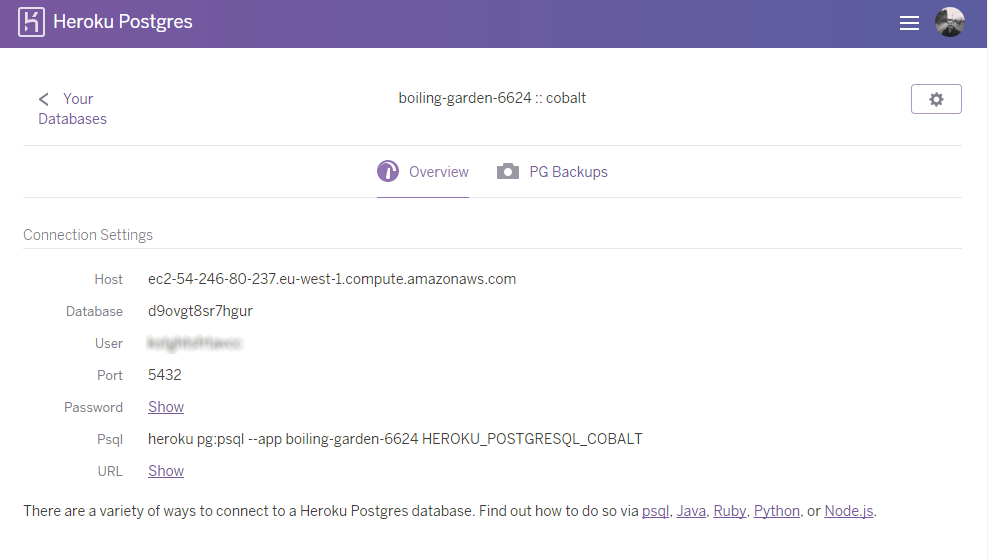**Detailed Caption:**

The screenshot depicts the interface of the Heroku Postgres software program, identifiable by the purple top bar spanning the width of the page, displaying its name and a distinct icon to the left—a white chair symbol combined with a lightning bolt. On the far right of this header bar, there is a menu button symbolized by three horizontal lines and an adjacent profile picture suggesting access to account information.

Centrally located on the white background of the main section, the text reads "boiling-garden-6624 :: cobalt". To its left, a "Your Databases" back button is visible, while a settings cogwheel icon appears to the right. Below this section, a horizontal line break separates the main screen content, followed by a navigation label "Overview" positioned centrally, alongside an eye icon. Next to this, the menu includes "PG Backups" accompanied by a camera icon, with "Overview" currently selected.

Further down, additional line breaks segment various sections starting with "Connection Settings". Within this section are fields labeled "Host" displaying a string of text characters, "Database" also with a string of text, "User" which is blurred out, "Port" indicating "5432", and "Password" which includes a clickable link to show the password, not currently selected. There is also a label for "PSQL" with associated text and numbers, and "URL" with another unselected link to display details.

At the very bottom of the interface, a text note provides guidance: "There are a variety of ways to connect to a Heroku Postgres database. Find out how to do so via psql, Java, Ruby, Python, or Node.js."